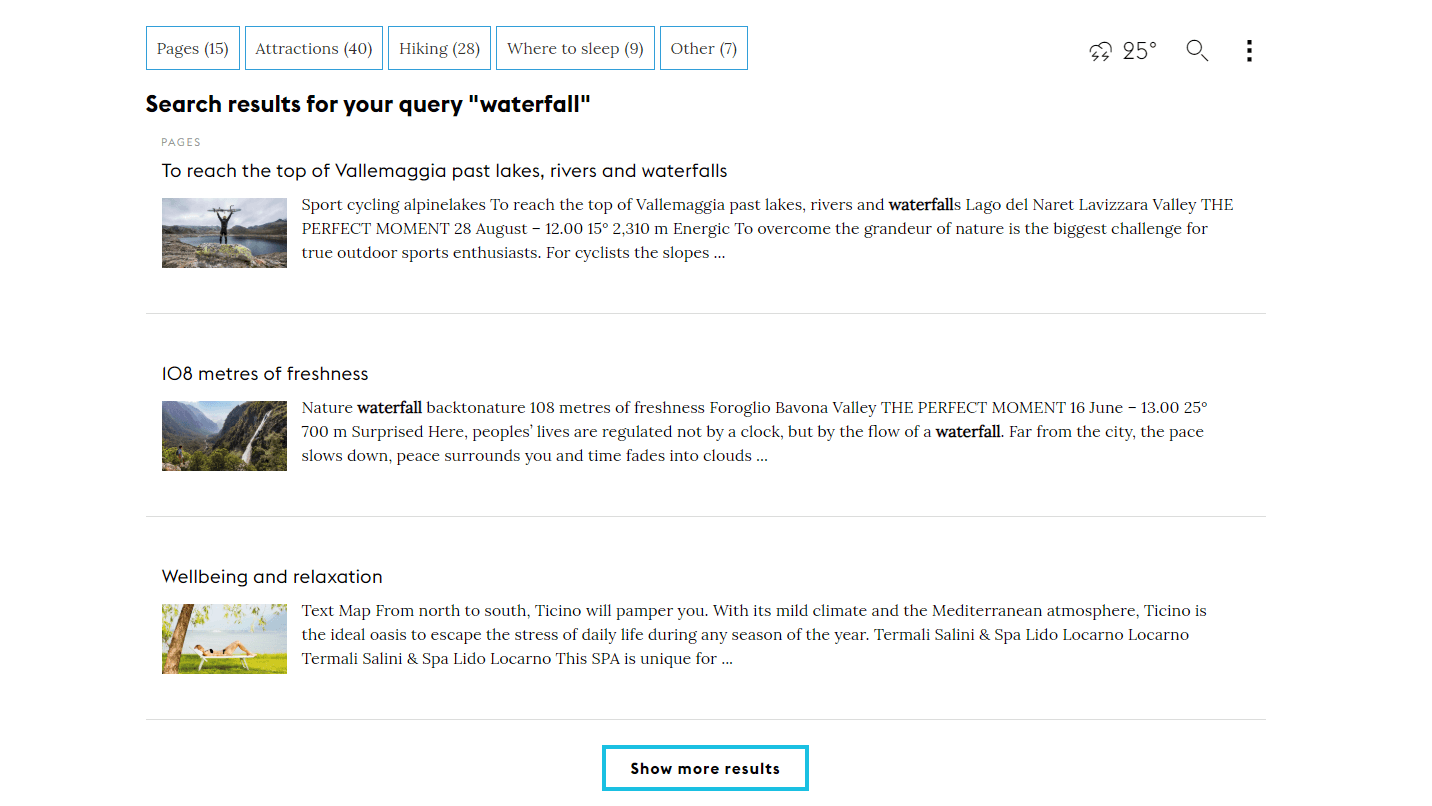Set against a solid white background, the image displays five buttons, each white with a blue outline. From left to right, the buttons are labeled: "Pages (15)," "Attractions (40)," "Hiking (28)," "Where to Sleep (9)," and "Others (7)." Below these buttons, large bold black text reads, "Search results for your query 'waterfall'." In very small gray text, the word "pages" can be seen.

The first search result features a description, "To reach the top of Alamajia past lakes, rivers, and waterfalls," accompanied by an image of a person standing on a boulder in front of a serene lake. The second search result highlights "108 meters of freshness, natural waterfall back to nature," with a location indicated as "Viroglia, Bavona Valley."